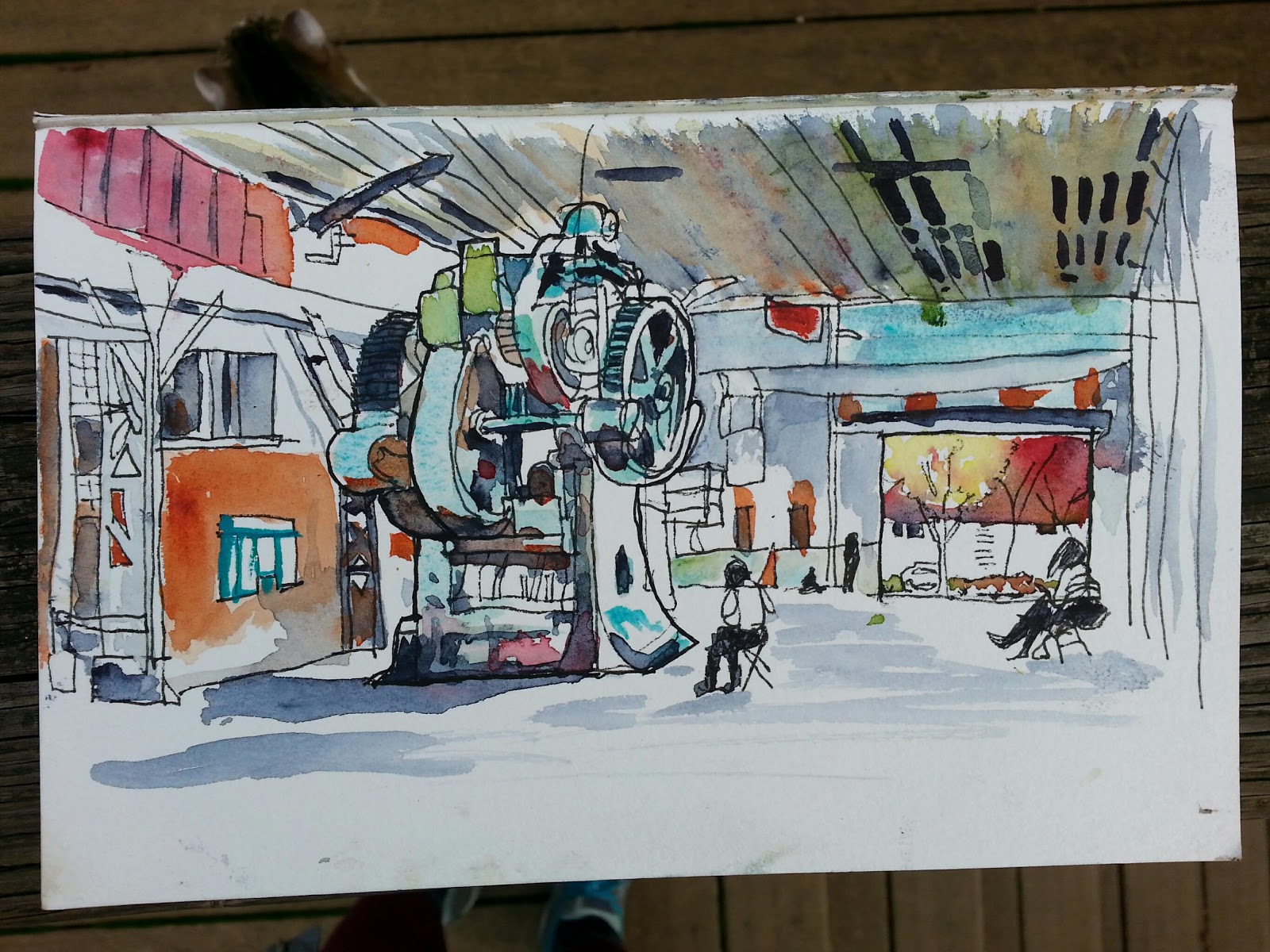This is a detailed watercolor painting displayed on a brown wooden wall, depicting a bustling machine shop. Dominating the center of the shop is an enormous piece of machinery adorned with an array of belts and wheels. To the right, two individuals sitting in black and white attire on folding chairs flank the machine—one directly beside it and another farther to the right. Behind this second person, a rolled-up door reveals an outdoor scene featuring a house with a red roof and two trees with bright autumn foliage—one with yellow leaves and the other with red leaves. On the far left of the composition, there's a door leading to another room, and a window adjacent to it. Above this door, red shapes are visible on the multicolored ceiling, which features a mix of browns, greens, and dark black stripes resembling possible holes. The entire artwork reflects a vibrant yet industrial ambiance, capturing the essence of a workplace with its vivid details and contrasting hues.